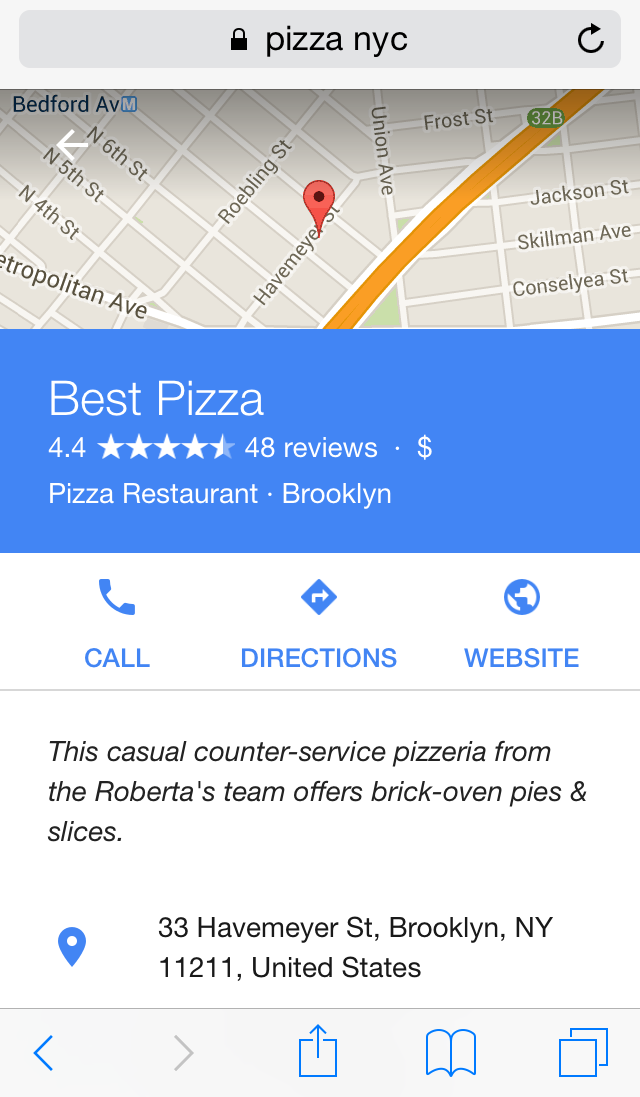In the midst of an emergency, discover Pizza Dots in New York City, highly rated with 4.4 stars from 48 reviews. Located at 33 Havemeyer Street, Brooklyn, NY, 11211, this casual, counter-service pizzeria is part of the Roboto's team. They specialize in brick-oven pies and slices, offering a delightful taste experience in a relaxed environment. For more information, you can call them, get directions, or visit their website.